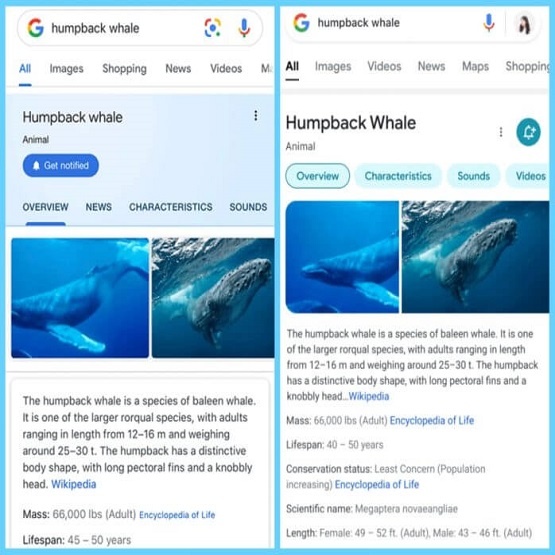The image depicts a structured search results page on Google, showcasing details about humpback whales. The background is a gradient of light blue, bordered on both sides by white rectangles.

On the left-hand side, there is a vertical menu bar with a gray outline, curving at the edges. This menu displays the Google "G" logo, followed by the text "Humpback Whale." Adjacent to these are multicolored symbols, a microphone icon, and the word "All" in blue, underlined by a short blue line. Below this line, navigation options such as "Images," "Shopping," "News," and "Video" are listed, though the last option is unclear. A grey line runs beneath these options, spanning the page's width. Further down, contained within a blue rectangle, the text "Humpback Whale, Animal" is visible. Adjacent to this, a blue button with a bell icon prompts users to "Get Notified." To the right, three black dots signify additional options. Below, navigation tabs labeled "Overview," "News," "Characteristics," and "Sounds" appear, underlined in blue when selected. Images of humpback whales and descriptive text are found beneath, with a reference to Wikipedia in blue and further informational writing below.

Mirroring the layout on the right-hand side, the Google "G" logo is again accompanied by "Humpback Whale," a microphone icon, and what appears to be a woman's face image. The word "All" is presented in black and underlined, followed by options labeled in grey: "Images," "Videos," "News," "Maps," and "Shopping." A similar gray line underscores these options. Additionally, "Humpback Whale, Animal" is displayed in a blue rectangle, followed by blue-outlined buttons for "Overview," "Characteristics," "Sound," and "Videos." More images of whales and extensive descriptive text are shown, with references to Wikipedia highlighted in blue and additional colored text interspersed with black text.